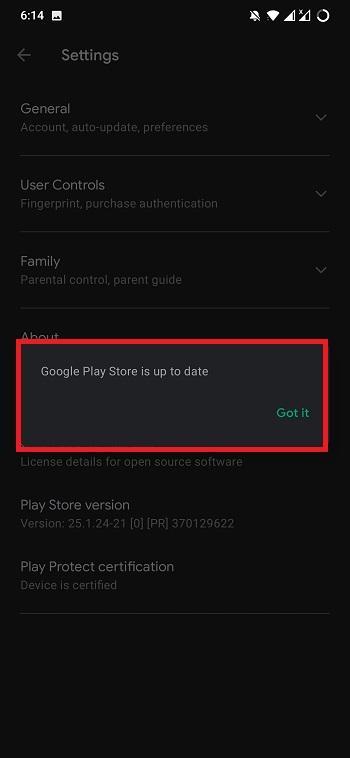This image is a screenshot taken from a cell phone, displaying a settings screen against a black background. At the top of the screen, the current time is shown in white numerals as 6:14. Surrounding the time indicator, a circular battery icon reveals approximately 75% battery life remaining. 

Various icons are positioned at the top of the screen. Below them, navigational text elements appear, including "Settings" with an arrow pointing to the left, followed by "General," "User Controls," "Family," and "About."

Prominently featured in the middle of the screen, a dark gray notification box with a red outline—almost giving it a glowing effect—pops up. The box reads, "Google Play Store is up to date," and includes a "Got it" button in green at the bottom right corner, which can be tapped to acknowledge the message.

Further down the screen, additional options are listed: "License details for open-source software," "Play Store version," and "Play Protect certification."